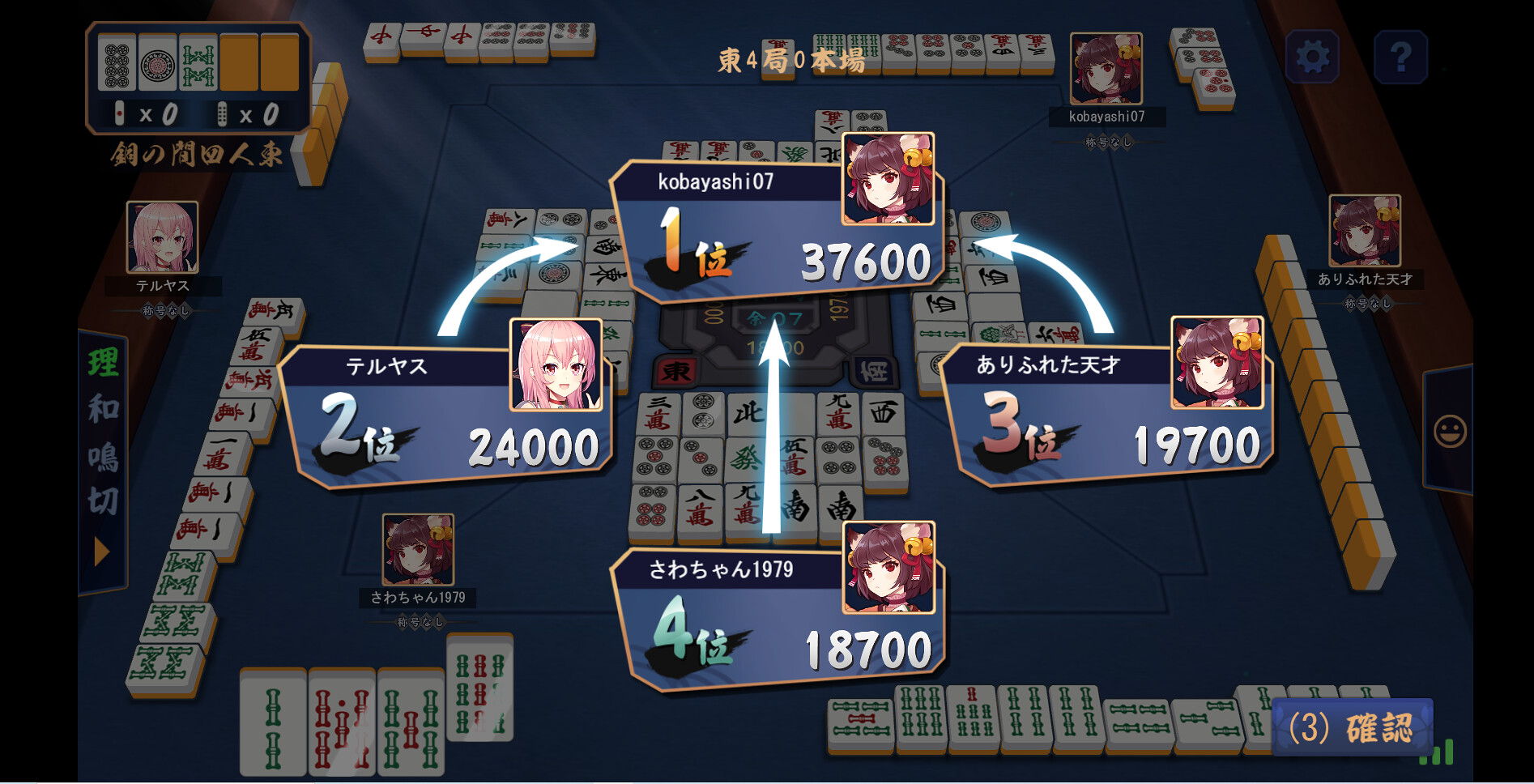This image depicts an intricate online Mahjong game, which is a digital version of the traditional, ancient tile-matching game. The screen showcases four manga-style avatars, each representing a different player with their respective scores. Three of these avatars feature Chinese characters as their names, while one also includes the year "1979" alongside the Chinese text. All arrows in the game interface point towards a fourth avatar positioned at the top, labeled "Kobayashi 07," a distinctly Japanese name. This indicates the game’s popularity in Japan, akin to other traditional games like Go. The scene highlights the cultural blend and competitive nature of this complex online Mahjong variant.